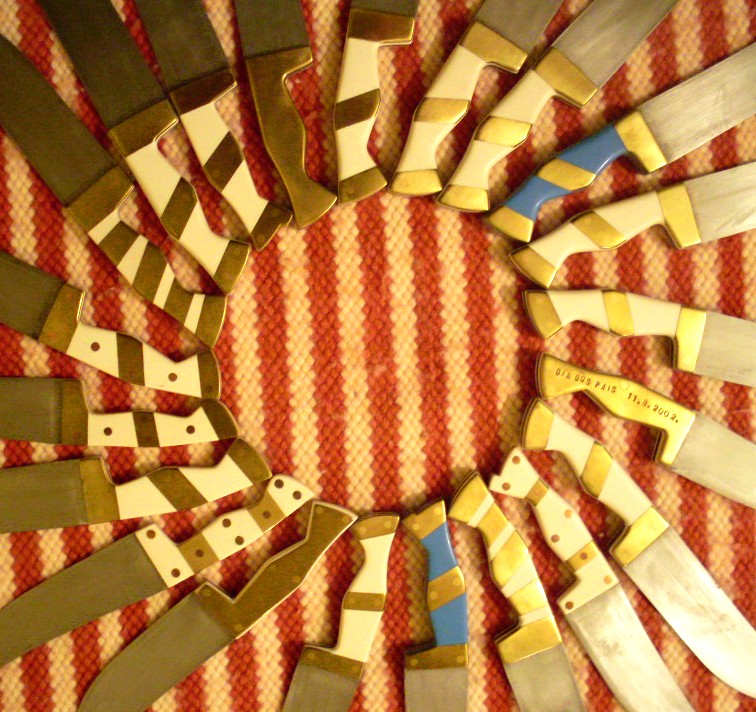The image features a striking arrangement of 21 knives meticulously placed on a cream and red striped towel. The knives are positioned in a perfect circle with their blades radiating outward, resembling the rays of a sun. Each handle points towards the center, forming a cohesive round shape. The handles exhibit a variety of designs: some are gold-outlined with wooden centers, others are white and beige, some have multiple stripes (ranging from two to four), and there are handles that are blue and gold, cream and gold, and brown with gold. One knife notably has an inscription reading "DOS Paris 11.3 202, 2002." Some handles are blemished with spots. The detailed diversity among the handles adds to the visual interest of this meticulously crafted display.